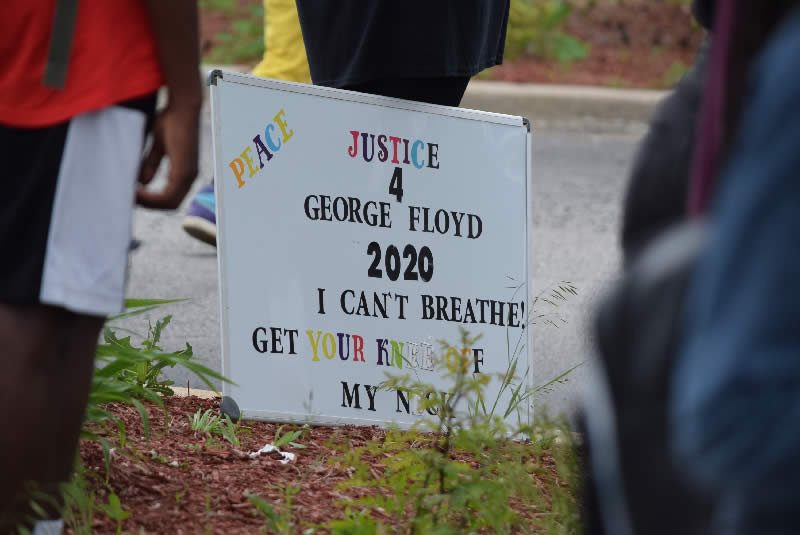The photograph captures a poignant scene from a Black Lives Matter march in 2020, centered around a handmade sign. The sign, fashioned from a whiteboard, bears an impactful message in all capital letters: "PEACE JUSTICE FOR GEORGE FLOYD 2020 I CAN'T BREATHE! GET YOUR KNEE OFF MY NECK." The text is a mixture of both black and vibrant rainbow-colored lettering, with certain words like "PEACE," "JUSTICE," and "YOUR KNEE OFF" highlighted in different hues. The sign rests on the ground amidst a gathering of people, though only their legs and partial torsos are visible. In the foreground, a small bush obscures the bottom portion of the sign, partially covering the text. This evocative scene underscores the urgency and emotional depth of the protest.